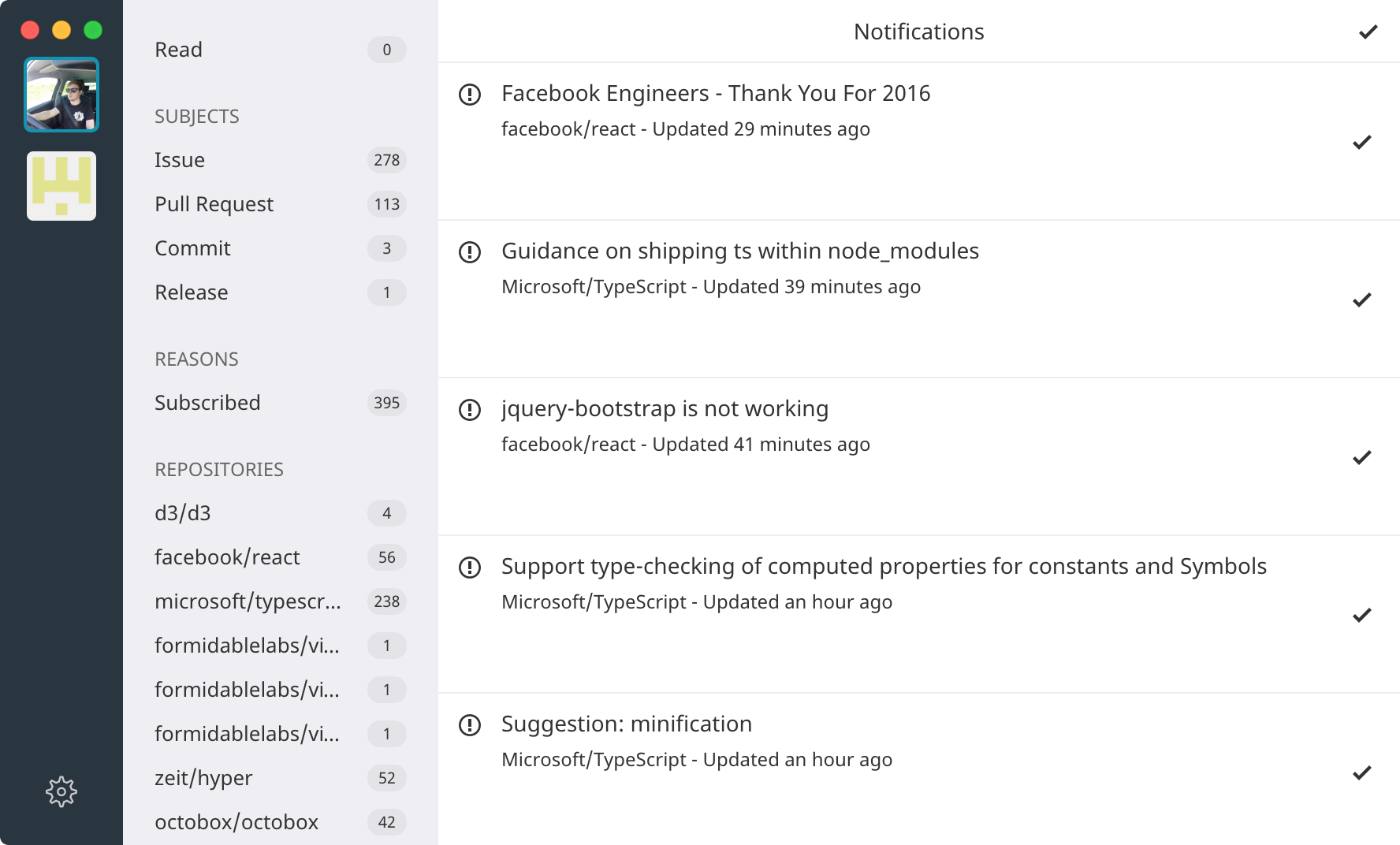The image displays a rectangular user interface segmented into two main columns. 

**Left Column:**

- The left column starts with a black vertical strip containing a set of colored dots: red, orange, and green at the top.
- Below the dots, there's a profile picture of a person.
- Under the profile picture, a white square features a logo in a yellowish-green color.
- Continuing downward, the rest of the column is predominantly black, culminating in a settings icon.
- The black segment is bordered by a shaded gray that completes the rectangular area.

**Right Column:**

- The right column is dedicated to notifications and is divided into five distinct sections.
  1. The first notification is titled "Facebook engineers guidance on shipping within node modules" and is followed by a timestamp indicating it was updated 29 minutes ago.
  2. The second notification reads "Query-bootstrap is not working" and was updated 39 minutes ago.
  3. The third notification, "Support type checking of computed properties for constants and symbols", has a timestamp of 41 minutes ago.
  4. The fourth notification states "Suggestion: Minification" and was updated an hour ago.
  5. The fifth notification, also updated an hour ago, is not named in the summary.
- Each notification section includes a checkmark to indicate completion.
- Beneath the primary text of each notification is a smaller line of print providing additional context specific to the update timestamp and content.

Overall, the image effectively organizes notifications and user settings within a visually structured interface.